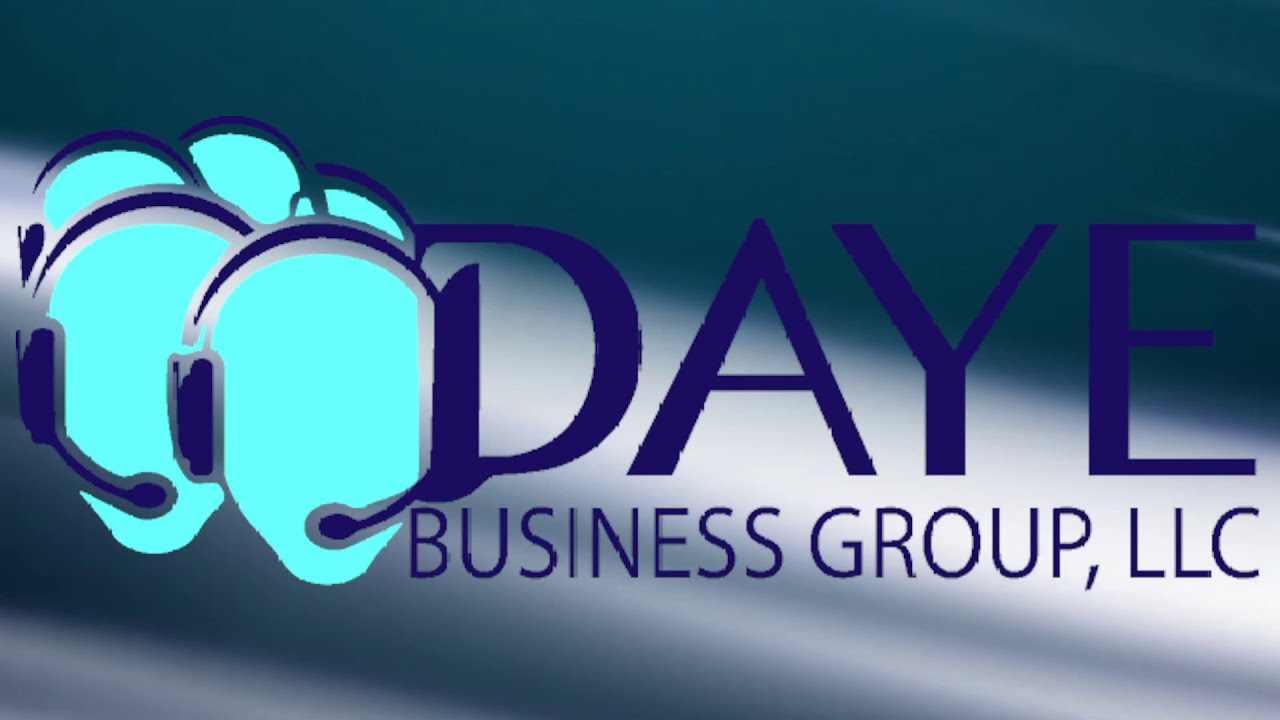The image displays a detailed graphical design of a business logo set against a background that mimics the side of a building with light rays cascading at a downward angle, casting shadows on the top and illuminating the bottom. To the left, the logo features the silhouettes of two customer service agents’ heads, both in solid light blue, with headsets and microphones adorning their heads. The first head’s microphone is on the right side, while the second head’s microphone is on the left. Behind these heads are three similarly light blue circles. To the right of these graphical elements, in thin black and blue all-caps font, is the company name "DAYE" with "D-A-Y-E" spelled out on the top line, and below it, "BUSINESS GROUP, LLC." The design has a blue background with a white streak cutting across the middle, giving the logo a professional and polished appearance indicative of a business consultancy.